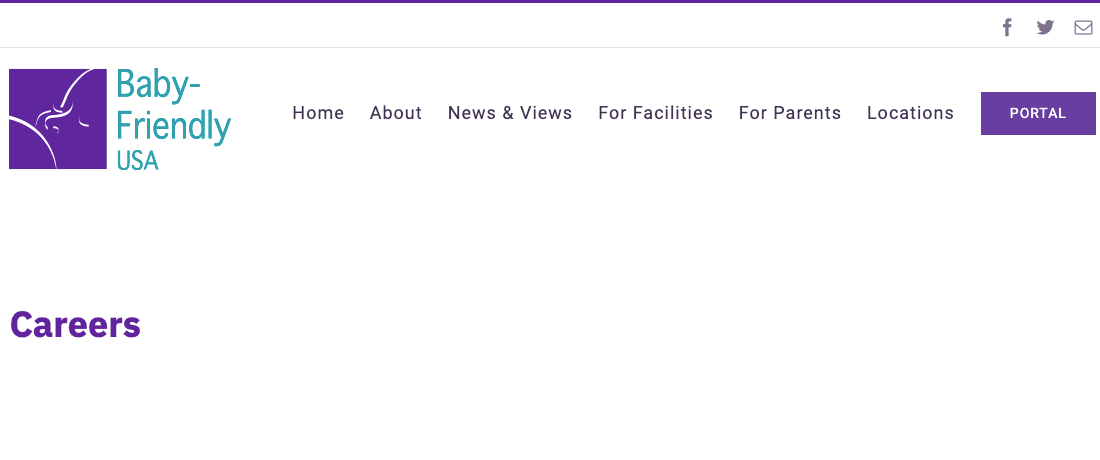At the very top of the image, there is a thin, horizontal purple rectangle stretching across the entire width of the page. Immediately below, on the right side, there are three icons in a slightly purple-gray color: a capital letter "F" representing the Facebook logo, a bird silhouette representing the Twitter or X logo, and an envelope symbol likely indicating an email option.

Directly beneath these icons, there is an even thinner horizontal gray line spanning the full width of the image. Below this line, on the left side, there is a purple square containing a white outline of a baby's face. Adjacent to this square, in a greenish-blue font, are the words "Baby-Friendly USA," with each word on a separate line and a hyphen connecting "Baby" and "Friendly."

To the right of this logo, there is a series of links displayed in a smaller purple-grayish font. These links include: "Home," "About," "News & Views," (where the "and" is represented by an ampersand), "For Facilities," "For Parents," "Locations," and finally, a purple rectangle labeled "PORTAL" in white capital letters. These links are laid out in a horizontal row, evenly spaced.

Further below, the word "CAREERS" is prominently featured in a larger, bold purple font similar to that used in the baby outline square. This text is left-aligned, adding emphasis to the section.